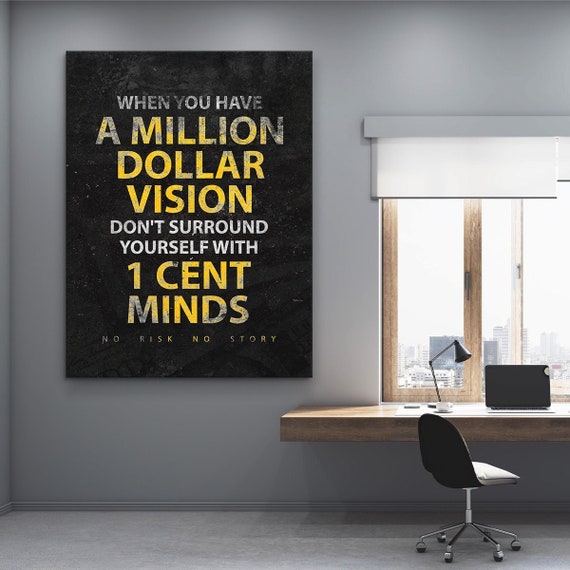In a minimalist grey office interior, the focal point is a large black-framed poster, almost the size of a window. The poster, crafted with a rustic gold and silver font, reads, "When you have a million-dollar vision, don't surround yourself with one-cent minds. No risk, no story." To the right of the poster, there is a window with a wooden frame extending outwards as a makeshift table, about five to six inches thick and extending two feet on each side. On this table rests an open laptop, a cup of coffee, and a black lamp with a movable arm. Below the table sits a sleek, black rolling chair with a leather back and seat, supported by a metal base with six wheels. The overall scene suggests a cozy yet motivational workspace, devoid of any people.